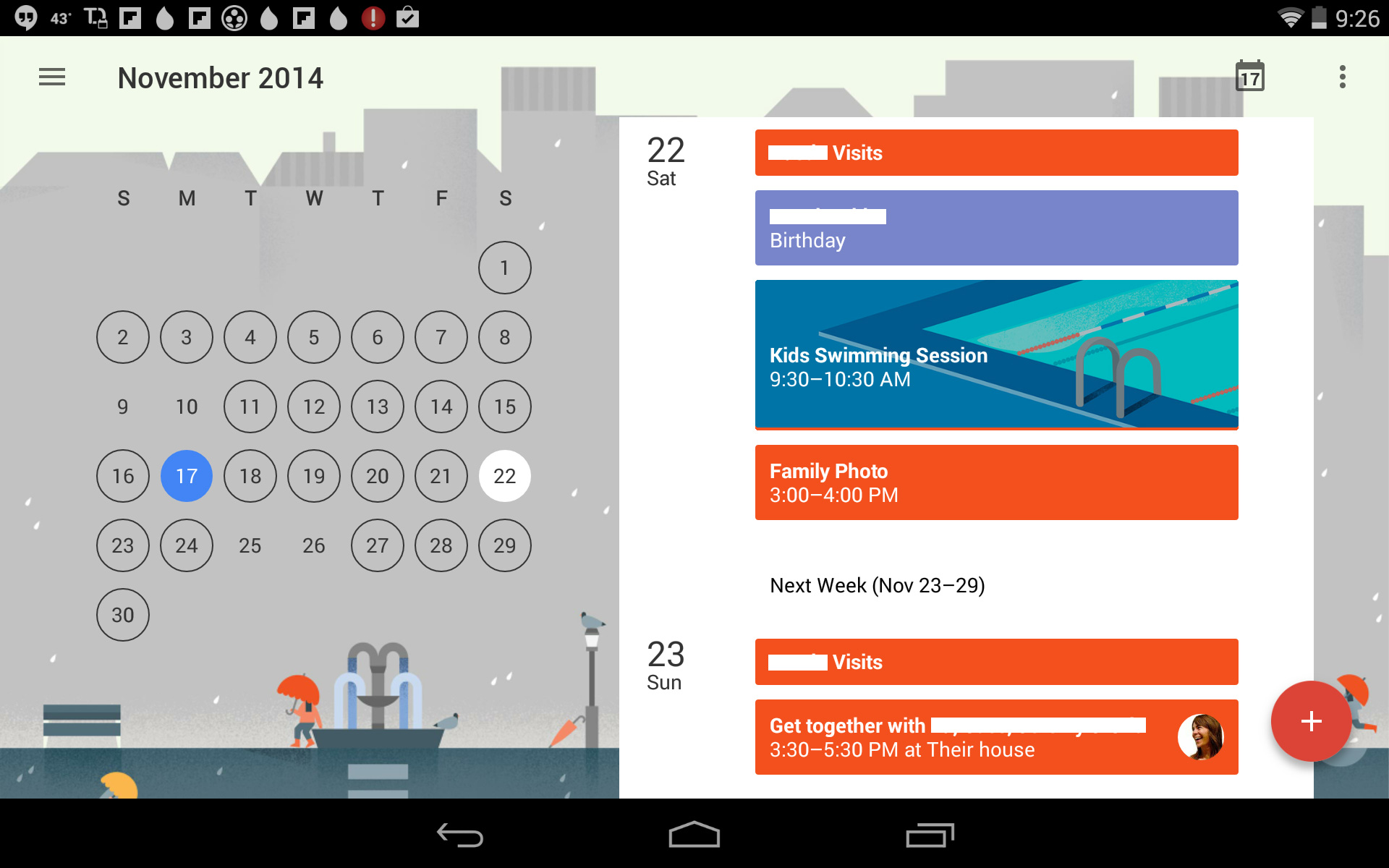The image showcases a smartphone interface displaying a calendar view. On the left half of the screen, the calendar for November 2014 is shown, with the entire month laid out against a grey background. The days of the week and dates are written in black, with each date enclosed in a circle. However, the circles for the dates 9 and 10 are not filled in. A blue circle highlights Monday, November 17, and another white-highlighted circle marks Sunday, November 22.

The right half of the interface has a white background. At the top left corner, "22 Saturday" is written in black. Below this, there's an orange header labeled "visit." The next section is titled "birthday," with a purple background. The calendar events are detailed as follows: 

- "Kids swimming session," scheduled from 9:30 to 10:30 a.m., with a background image of a swimming pool.
- "Family photo," set for 3:00 to 4:00 p.m., set against an orange background.

At the bottom of the section, there is a link for "next week November 23 to 29," on a white background. The events for the following week begin with a "visit" on Sunday, November 23, noted on an orange background, followed by a "days get together" event from 3:30 to 5:30 p.m. at the house, also on an orange background.